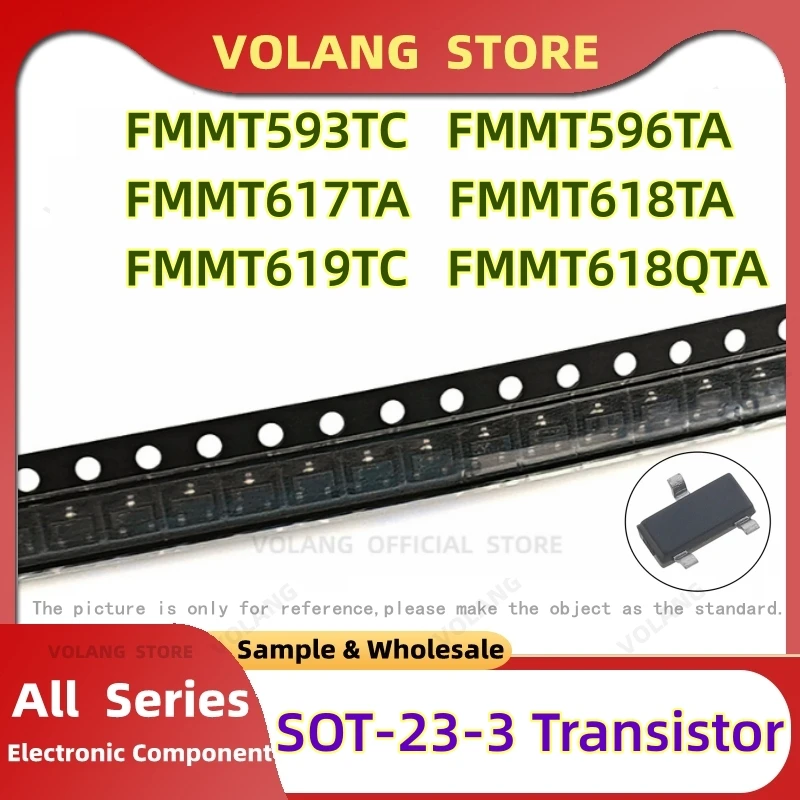This square-shaped image, measuring approximately 6 inches by 6 inches, appears to be an advertisement for electronic components. It features a prominent red border that encircles the entire image, with the top portion dipping down in the center, highlighting the store’s name in large, yellow letters that read "Bowling Store". 

Below the store name, six rows of serial numbers are displayed in bold, black print with a greenish-yellow outline; each begins with the letter sequence "FMMT" followed by unique variations such as "593TC", "596TA", "617TA", "618TA", "619TC", and "618QTA". 

A black ruler-like strip with white holes runs horizontally across the image, dividing the content. 

In the lower section of the image, the left corner features a text box with a red border that bubbles out toward the right. Inside, white print reads "All Series Electronic Components". Adjacent to this, towards the right, is a thin yellow oval with black print indicating "Sample and Wholesale." Below this oval is a description in purple print with a yellow outline, specifying "SOT-23-3 Transistor."

Toward the lower part of the image, there is also a depiction of circuitry, along with a circle containing a small circuit board. The text "Volang Official Store" is present alongside a disclaimer that states, "This picture is only for reference. Please make the object as a standard."